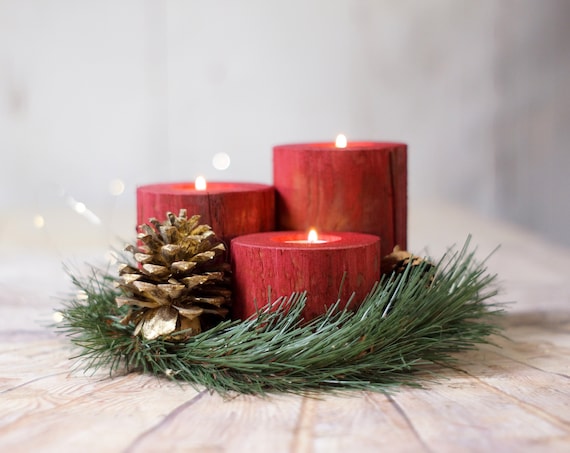This festive image features a Christmas-themed candle arrangement centered on a pale wooden table. Dominating the scene are three vivid red candles of different heights, each with a small, glowing flame. The shortest candle is positioned in front, with progressively taller candles behind it. Encircling these candles is a lush green wreath adorned with pine needles, ferns, and a golden pine cone visible to the left. The candles appear to have textured bodies with subtle lines and could be either solid wax or wooden holders with tea lights. The background is a soft gray, slightly blurred, ensuring that the focus remains on the detailed and colorful centerpiece. Small glittery accents are vaguely noticeable in the arrangement, adding to the festive charm.